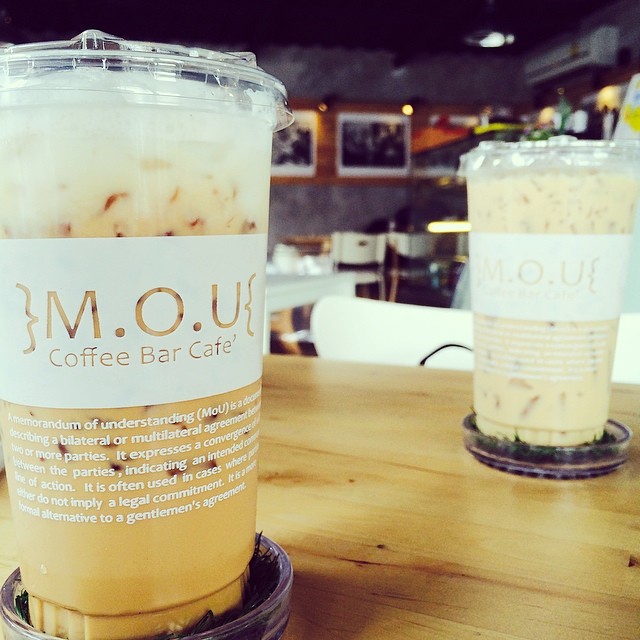The image captures a cozy scene inside MOU Coffee Bar Cafe. At the center of the natural wood table, there are two plastic cups prominently featuring the cafe's logo. The cup closest to the camera contains a light brown coffee drink, possibly a cold brew, while the other cup holds a milky iced coffee. Both drinks are brimming with ice. The label on the cups includes an extensive text description about a memorandum of understanding, though it is partially obscured. Surrounding the table, the cafe's inviting interior unfolds: a series of tables and chairs, a gray wall, and a black ceiling. A section of the wall is adorned with black and white photographs mounted on a wooden panel, and an AC unit is visible in the upper right corner, adding a touch of modern comfort to the space.